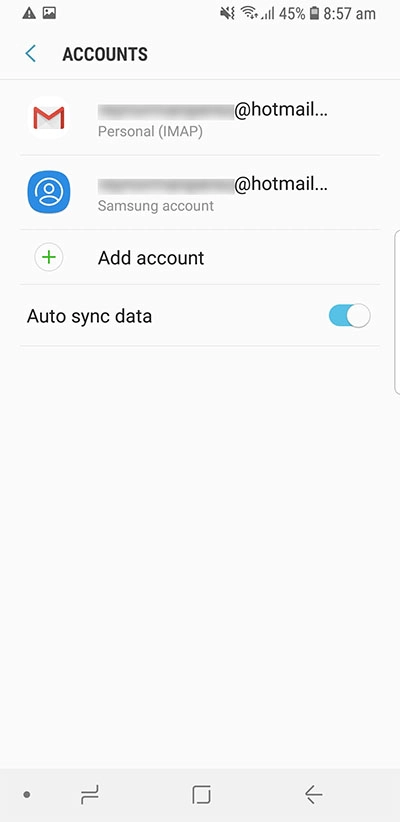The image depicts a mobile application interface that allows a user to manage multiple email accounts across different email service providers. One section of the interface shows a Gmail icon associated with a Hotmail email address, indicating that the user has added their Hotmail account to the Gmail app, enabling them to access and manage their Hotmail emails within the Gmail client. Additionally, another Hotmail account is visible in a separate email app, possibly a Samsung email client, which allows for multiple email accounts to be configured. There is an "Add Account" button, suggesting that the user can add more email accounts if needed, and the "Auto Sync Data" feature is toggled on, ensuring that the emails are kept up to date automatically. This interface serves as a centralized hub for managing different email accounts across various apps and services.